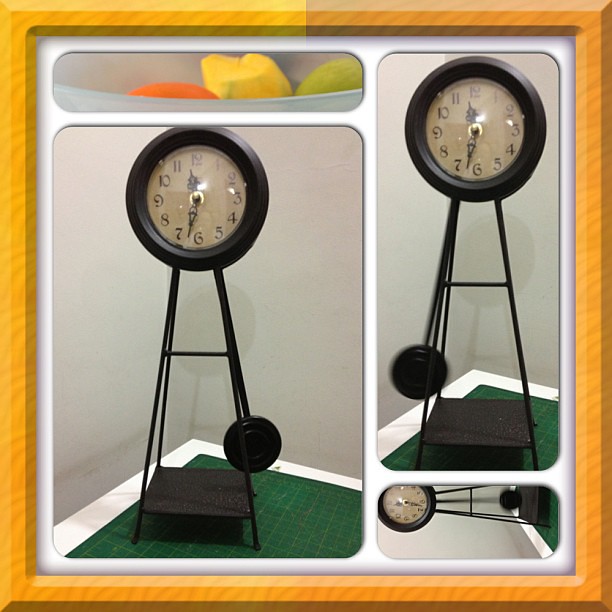This framed collage-style image consists of four photographs matted into different sections, each depicting a grandfather-style pendulum clock in varying positions. The frame itself transitions from brown at the center top, gradually lightening to yellow as it moves to the right, down, and then back up. The primary photo occupies a large rectangular section, showcasing a clock with a thick, round, brown frame reminiscent of a small car wheel, housing a glass-covered ivory placard with black Arabic numerals. The clock's hands point to 11:33, and it stands on a black tripod with four legs, set upon a green, gridded cutting board against a white wall. The pendulum in this main image is to the right. Adjacent to it, another image depicts the same clock with the pendulum to the left. At the bottom, a slightly smaller sideways image shows the pendulum centered. An additional, smaller section at the top contains an unclear depiction of orange, yellow, and green objects. The entire collage appears to be AI-generated.